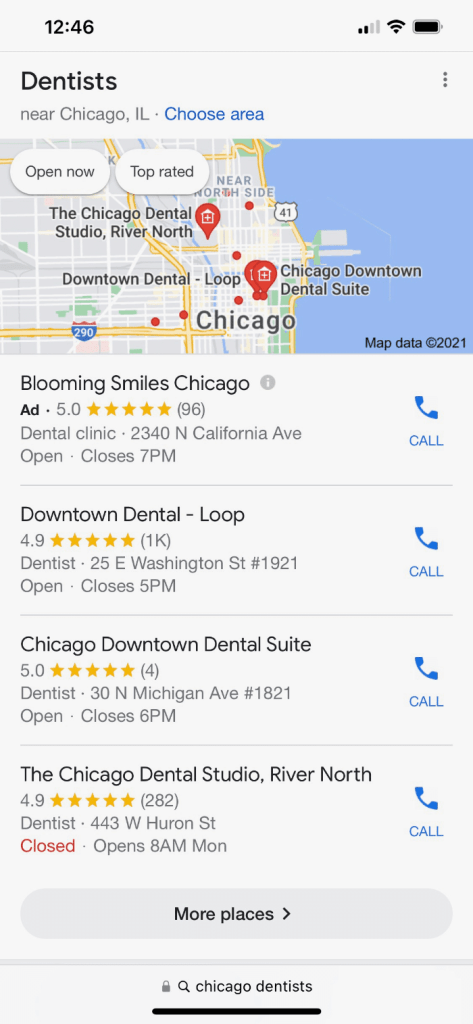The image displays mobile search results for dentists near Chicago, Illinois. At the top of the screen, the time, battery level, and connection information of the phone are visible. The search query "dentists near Chicago, Illinois" is prominently displayed. Below the query, there is a blue hyperlink labeled "Choose area." A small map with red markers indicates various dental locations.

Underneath the map is a list of four different dental establishments. Each entry includes the name of the establishment, its Google rating, the type of facility (whether a dental clinic or dentist), the address, current status indicating if it is open, and the closing time. To the right of each entry, there is a blue phone icon with the word "Call" beneath it, enabling users to quickly contact the businesses.

At the very bottom of the search results, there is a button labeled "More places," allowing users to load additional search results.